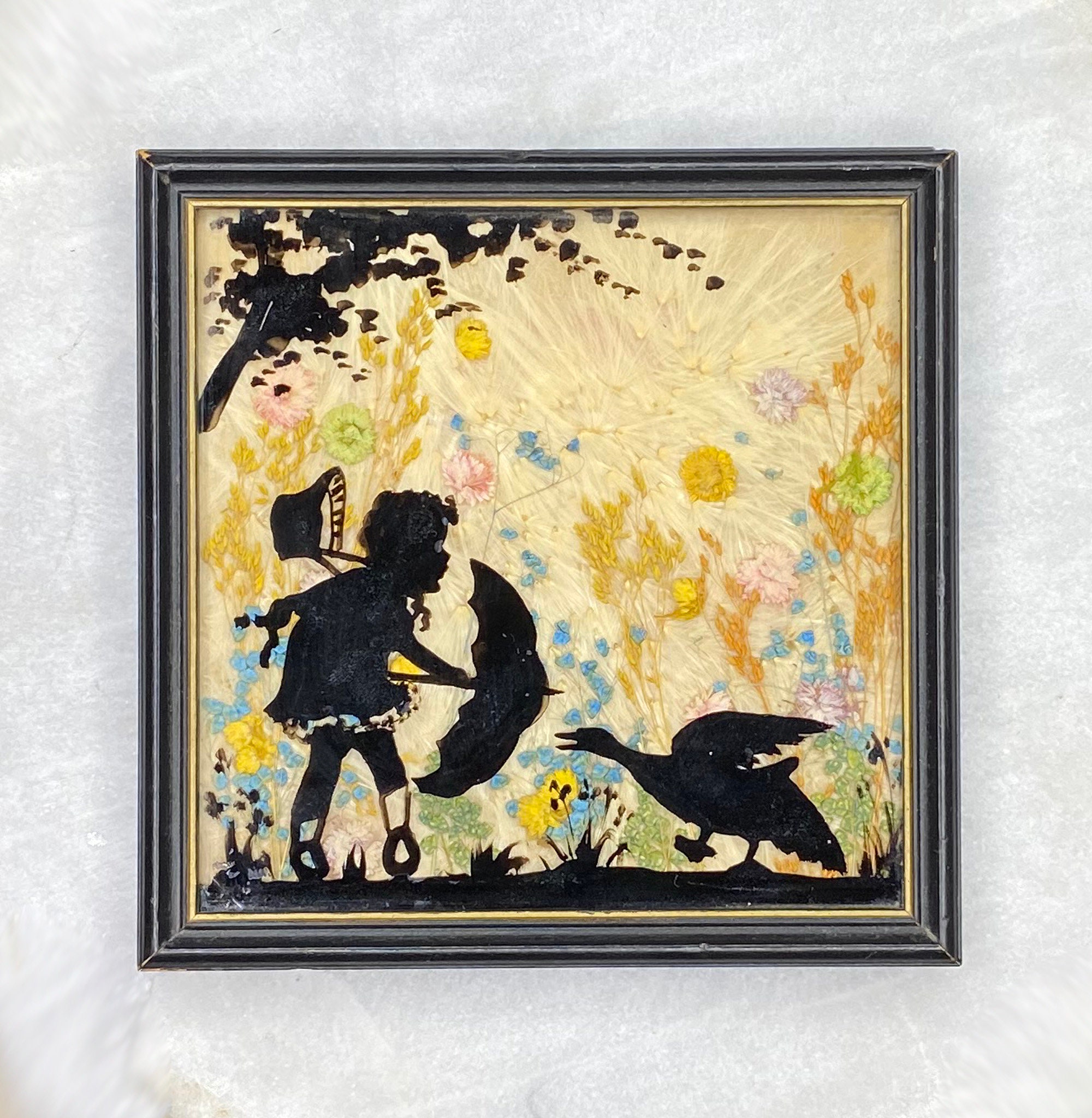The image captures a framed painting with a dark gray wood frame and a gold liner. The central scene is a silhouette featuring a young girl and a goose, both rendered in black against a cream-colored background. The girl, positioned on the left side, is seen in profile with her bonnet trailing behind her as she points an open umbrella toward the right side, where a goose is aggressively approaching with its beak open and one foot raised. Above the pair is the silhouette of a tree, while beneath them, the ground is also depicted in black. Flanking the composition are tall, gold stalks of grass or flowers, adorned with additional plants and flowers in hues of yellow, green, pink, and blue, creating a vibrant contrast against the cream background. The overall effect is an engaging interplay of color and silhouette, capturing a dynamic moment in a scene that exudes both whimsy and tension.